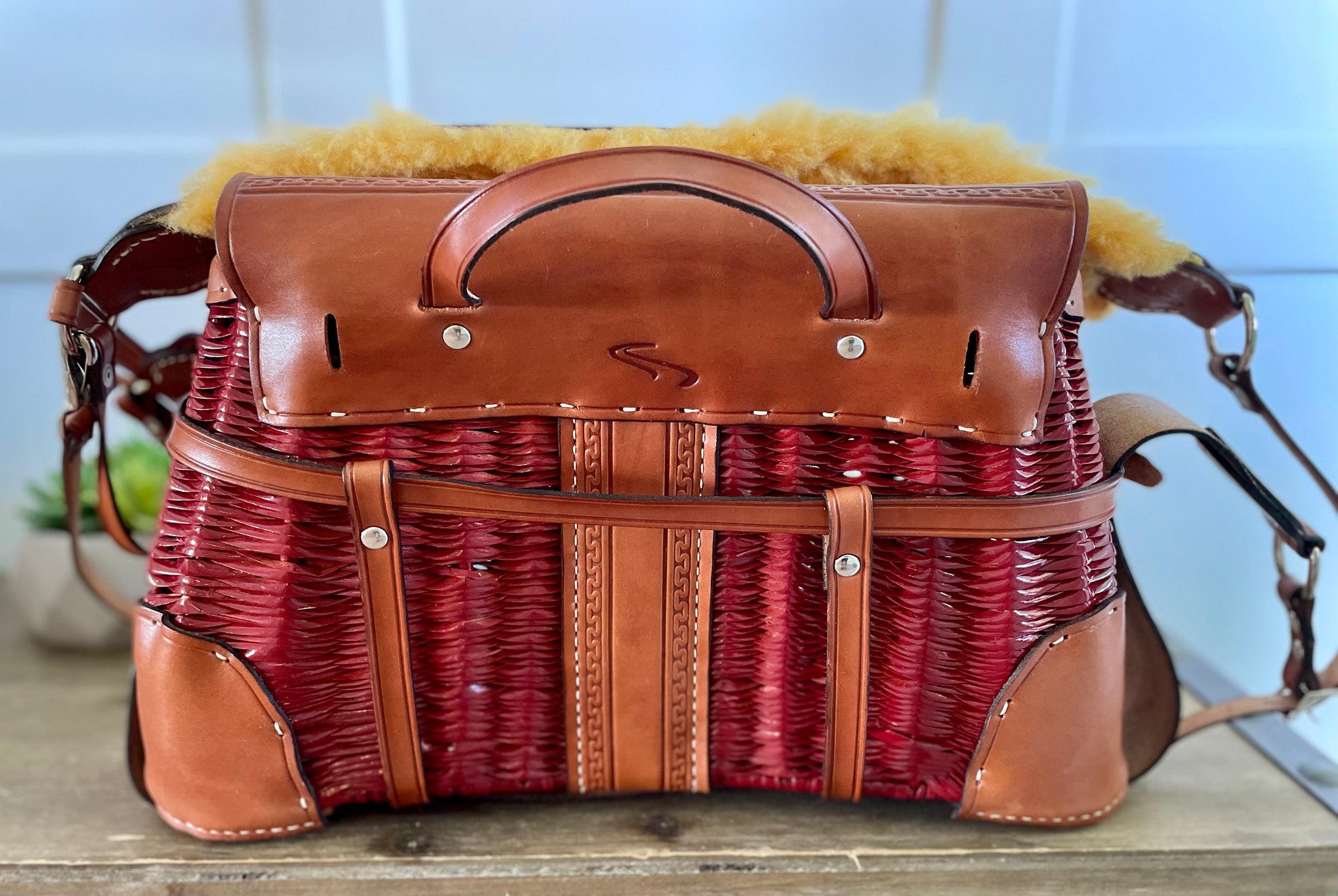This image showcases a unique and beautiful designer handbag prominently displayed on a light gray, wood-textured table with a gray metal edge border. The background features a bluish-white wall with molding, which is slightly blurred to keep the focus on the purse. Nearby, a succulent plant in a stone bowl adds a touch of natural decor to the setting.

The handbag itself is the centerpiece of the image. The body of the bag is made of a woven red wicker material, giving it a basket-like appearance. The purse's corners are reinforced with meticulously hand-sewn light brown leather patches that cover about a third of its height, ensuring durability and aesthetic appeal. Two leather harnesses wrap around the bag, securing a central leather band in place.

The purse features both a soft, yellowish sheepskin shoulder strap, designed for comfort, and a practical leather handle for versatile carrying options. The closure of the bag is a brown leather flap with a distinctive carved arrow logo, suggesting it might be the manufacturer's mark. Overall, this handbag combines vibrant materials and textures, making it both a fashionable and functional accessory.